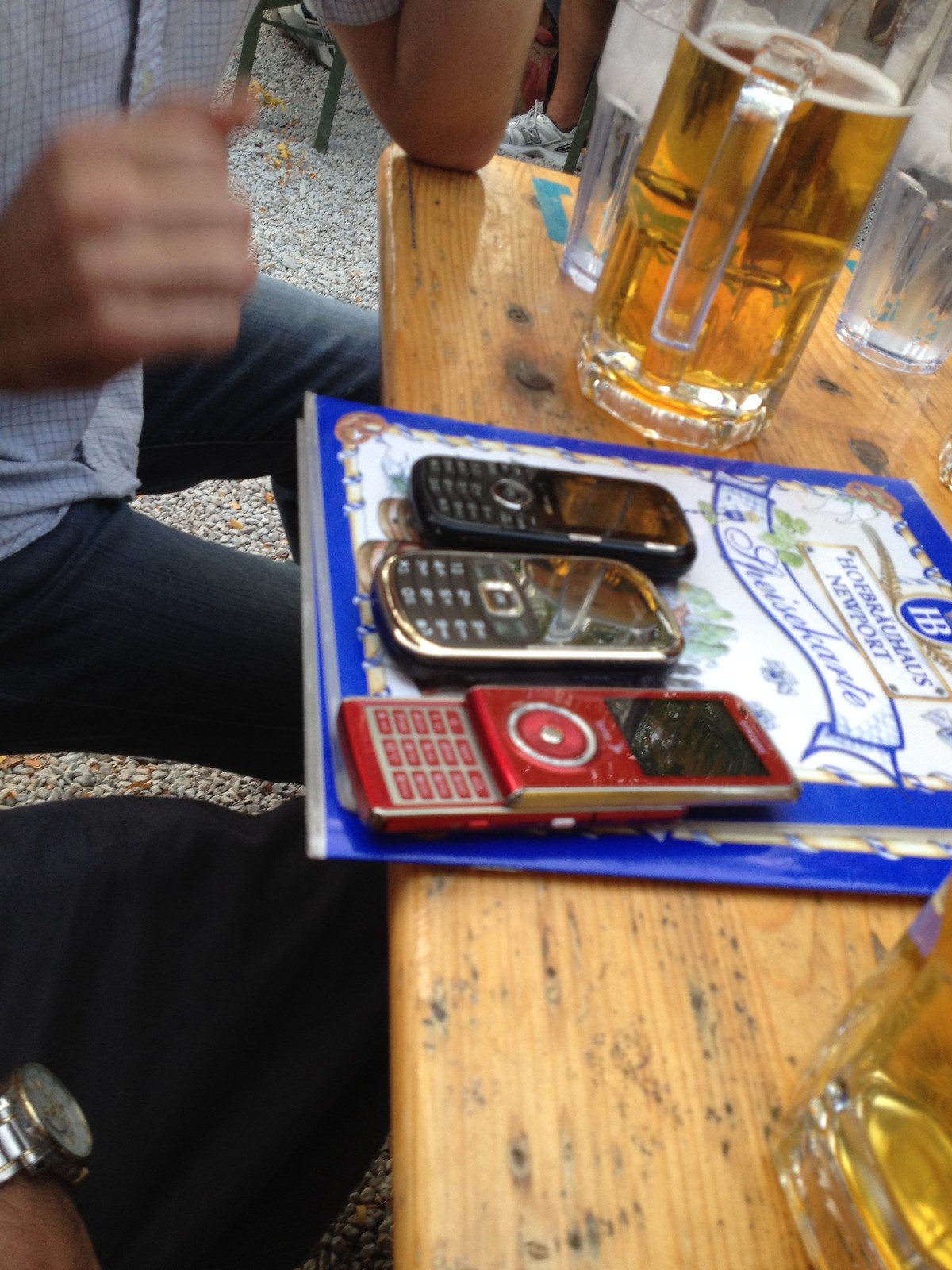The photograph captures a moment at an outdoor wooden table bathed in bright sunlight. Two men, identifiable by their black pants, are seated at the table with their arms and elbows resting on it. In the foreground, there are several mugs of beer, with one prominently positioned at the top right corner and another just glimpsed at the edge of the frame. Also on the table stand glasses of water, contributing to the relaxed, convivial atmosphere.

At the center of the table lie two stacked blue and white menus, hinting at a possible German locale with partially legible text that reads, "Knopfbrauch Newport." Adding a touch of nostalgia, three early 2000s cell phones are placed atop the menus. The phones include a bright red slider phone, a classic black phone with brass trim, and a gray model, all of which gleam under the sunlight despite one screen being cracked. Below the table, a shoe attached to a leg is visible, further emphasizing the casual setting.